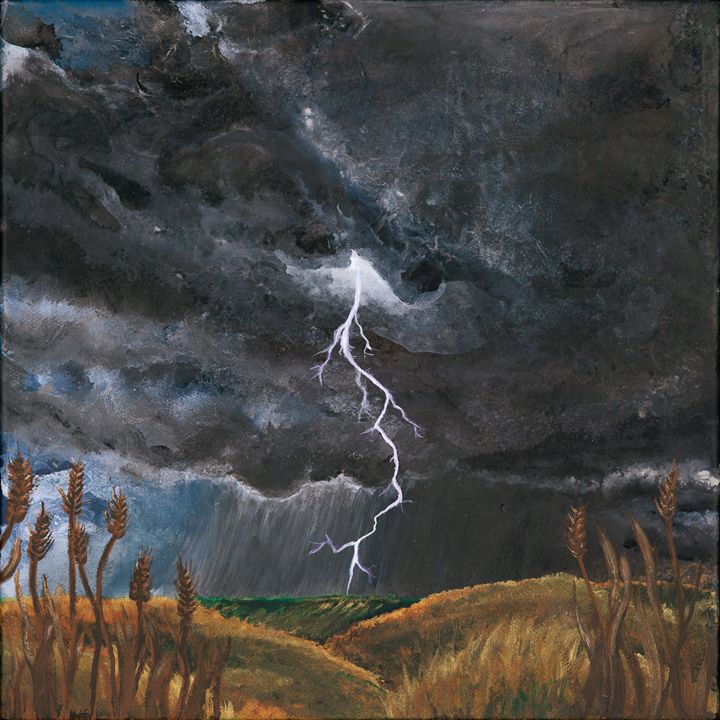The image is a detailed painting that depicts a stormy day in a field. Dominating the top half of the painting are dark, ominous black and gray clouds. Rainfall is represented by straight gray lines cascading down from these clouds. A brilliant white bolt of lightning flashes dramatically from the center of the storm clouds, striking the green grassy ground below. The lightning strike, positioned centrally, is the focal point of the painting. The background reveals green grass, while the foreground features two hills colored in shades of brown, orange, and yellow, reminiscent of hay or grassy mounds. Tall, wispy wheat plants adorn the bottom corners of the painting. Despite the painting having a texture similar to charcoal, it incorporates various colors, suggesting the use of colored charcoal or a mixed media approach. The scene vividly captures the impending storm's advance towards the tranquil wheat field, highlighting the contrast between the dark, turbulent sky and the serene landscape below.